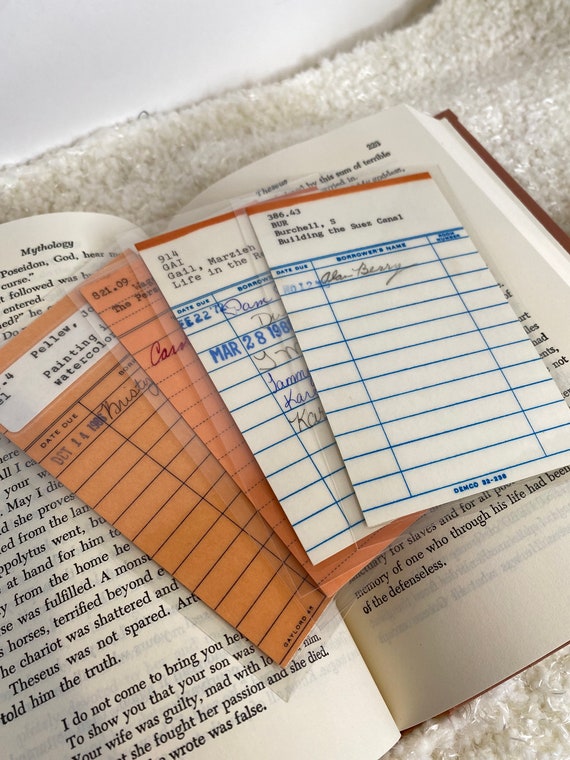This photograph captures a serene indoor scene featuring an open book resting on a softly textured, fuzzy white blanket. The book is open to a page brimming with text, with the heading "Mythology" indicating a passage about Poseidon. Lying atop the book are four rectangular library cards or borrowing slips, fanned out in a neat, overlapping arrangement. These cards—two white and two orange—display columns and rows formatted for recording borrowers' names and other details. The book beneath these slips appears to be in pristine condition. In the background, a pristine white wall adds to the overall calm and minimalistic aesthetic of the composition.